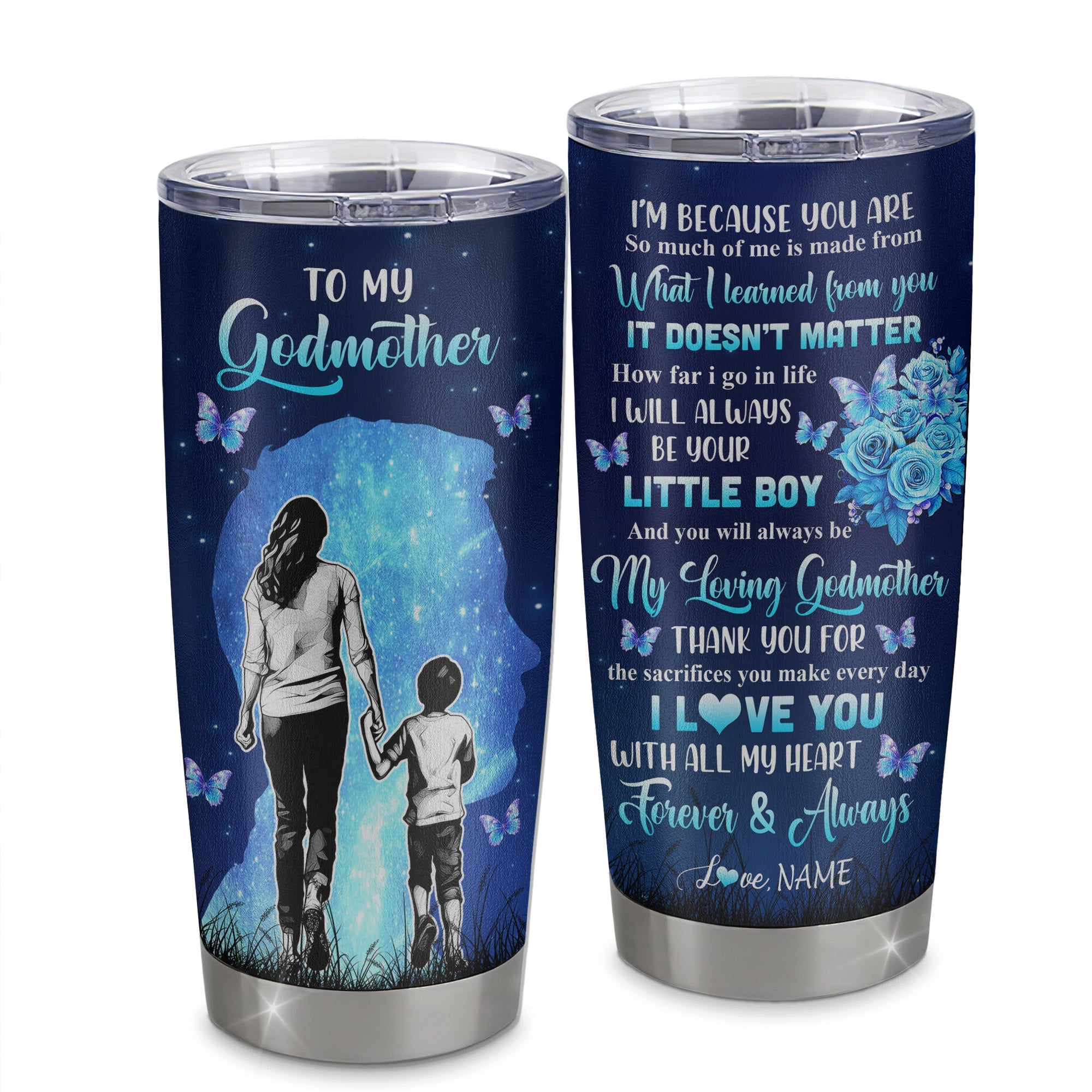This image showcases a stainless steel insulated tumbler, designed as a heartfelt custom gift. The tumbler features a dark navy blue background that gradually transitions to a lighter blue towards the bottom, with a stainless steel silver base. The top is fitted with a clear acrylic or hard plastic lid, ensuring the contents stay cold.

On the front, at the top, the text "To My Godmother" is prominently displayed in cursive white lettering. Below this inscription, there is a detailed design. It includes a light blue silhouette of a boy's profile, overlaid with a black and white illustration of a woman with long hair holding a child's hand. The two figures are depicted from behind, walking on grass, with the woman gazing up into the stars while the boy looks down. Surrounding them are four butterflies in shades of blue and purple, adding a whimsical touch to the scene.

The back of the tumbler carries a deeply personal message in an array of fonts, including script and cursive, in blue and white lettering. It reads: "I’m because you are. So much of me is made from what I learned from you. It doesn’t matter how far I go in life, I will always be your little boy, and you will always be my loving godmother. Thank you for the sacrifices you make every day. I love you with all my heart, forever and always." Spaces are provided for adding a personalized sign-off with the giver's name. The text is adorned with blue butterflies and roses, further enhancing the heartfelt nature of this gift.

Overall, this tumbler serves as a beautiful and functional keepsake, ideal for showing gratitude and affection to a beloved godmother.